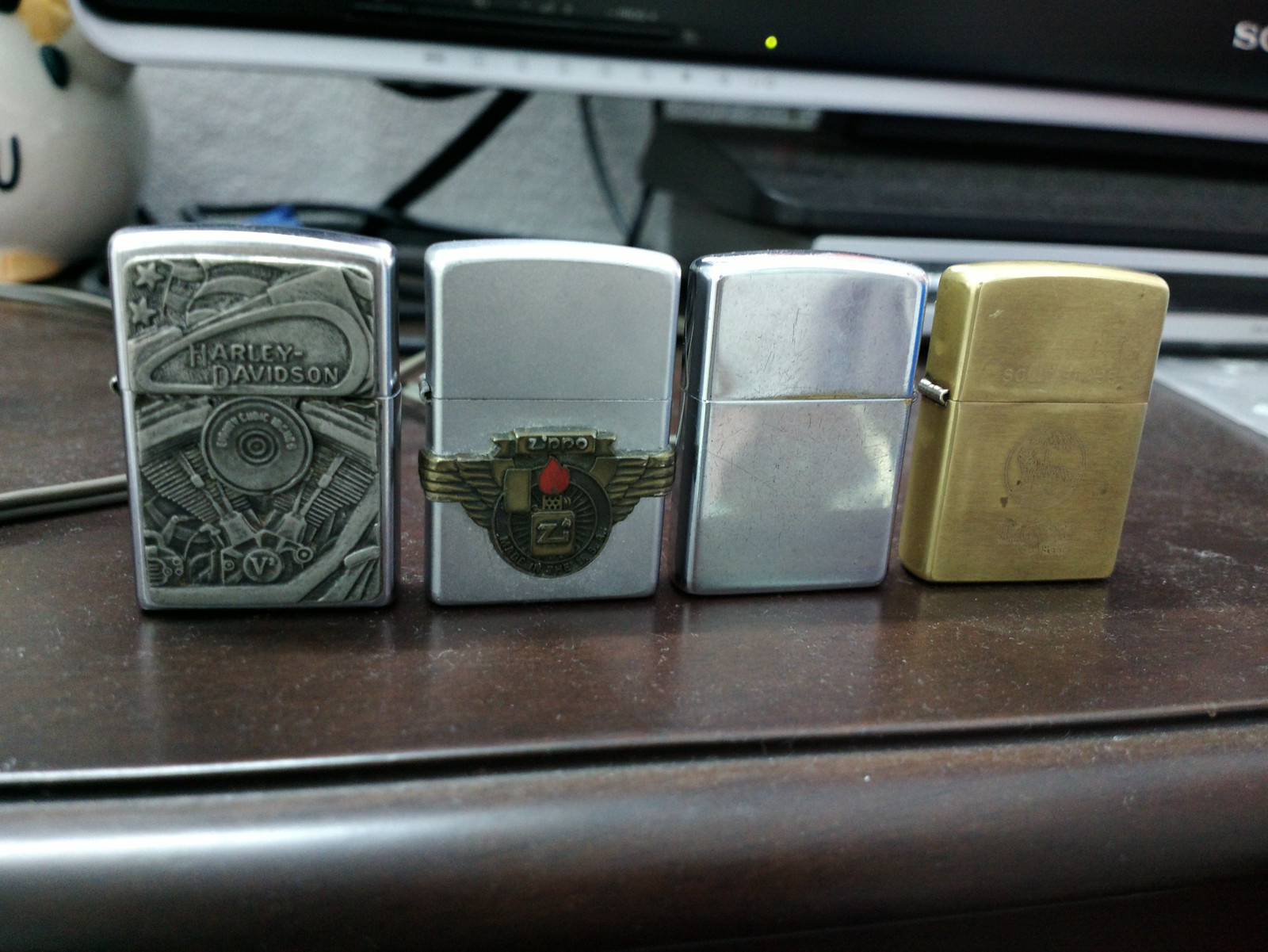This photograph captures four distinct Zippo lighters in a row, elegantly displayed on a dark brown wooden table. From left to right, the first lighter features intricate carvings depicting a Harley-Davidson motor, with the brand name emblazoned across the top lid. The next lighter sports a metallic badge with wings extending from either side of a circle, accompanied by the Zippo logo at the top; the emblem is highlighted with a touch of red where a flame would appear, giving it a unique character. The third lighter stands out with its sleek, polished silver finish, free from any additional adornments. The final lighter gleams in a solid gold hue, showing signs of use yet maintaining its luster.

In the background, the very bottom edge of what appears to be a Sony television or computer monitor is visible, identifiable by a partial "S". Scattered wires lie on the table, adding a touch of realism to the setup. Additionally, there is a black keyboard and a segment of a black computer. On the far left, a white object with a distinctive black circle and a yellow spot can be seen. The entire scene is set against a backdrop of a white wall, providing a neutral contrast to the rich, dark wood and the gleaming metallic surfaces of the lighters.